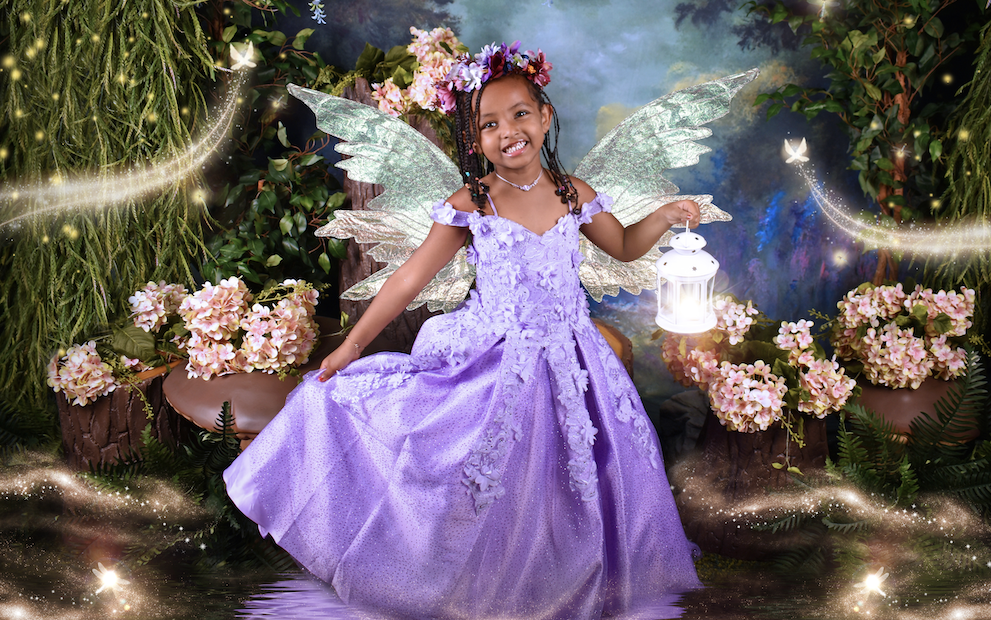This enchanting photograph captures the magical scene of a young African-American girl, dressed as a fairy, standing centrally against a whimsical forest backdrop. The setting is adorned with lush greenery on either side with pale pink or peach flowers nestled among the dark brown tree trunks, all shrouded in a touch of mysterious fog. The ground appears to be dark earth, evocative of a woodland floor. The girl, with her radiant smile, stands in the foreground, her brown skin glowing. She wears a lovely lavender purple dress embellished with floral appliqués and sparkly accessories, including a shimmering necklace. Her hair is styled in charming braids adorned with small colorful beads. On her head, she wears a feather crown, and on her back are delicate fairy wings, likely made of paper mache. She holds a bright white lantern that adds a touch of enchantment to the scene. Flitting around her are magical butterflies with glittery golden streams of light following their paths, while pixie dust sparkles throughout the image, enhancing the fairy tale atmosphere. The composition includes whimsical elements like fake stumps and plants, as well as cherry blossoms and mushrooms, creating a dreamlike, fantasy setting reminiscent of a fairy godmother's enchanting realm.